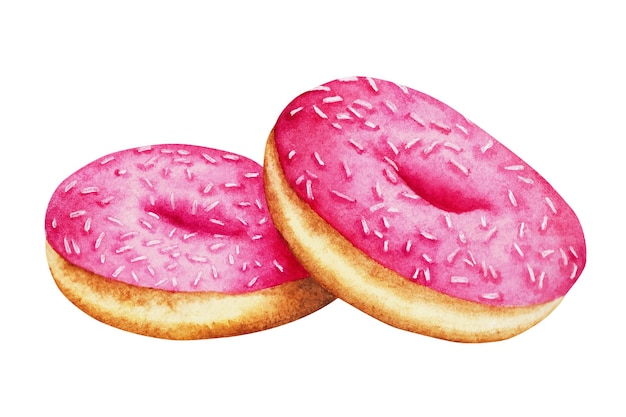The image features two artistic, digitally or ink-drawn donuts set against a plain white background. The donuts are round with holes in the middle, having a brownish hue and light tan-yellow edges. They are adorned with a layer of pink frosting covering the top and upper third, sprinkled with white sprinkles. One donut is positioned flat on the surface, while the other is angled slightly on top of it, giving the impression of stacking. The donuts have a thin, bagel-like appearance rather than the typical plump form. The image is simple, devoid of any text or additional elements, focusing solely on the two donuts.